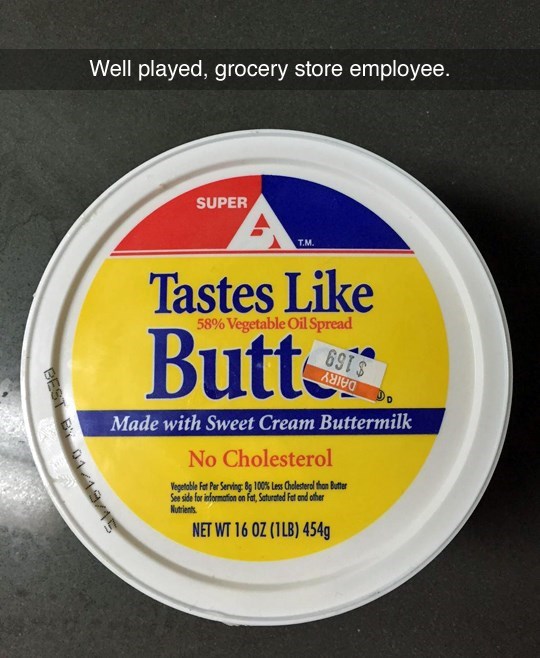This image, likely taken with a mobile device, features a white, round, plastic container of butter prominently labeled with a humorous oversight. The top of the image includes the caption, "Well played, grocery store employee." The container's lid is adorned with a blue, red, and yellow icon, punctuated with a label that partially covers the word "butter," resulting in the phrase "tastes like butt" instead of "tastes like butter." The label on the lid reads: "Tastes like butter, made with sweet cream buttermilk, no cholesterol," and further details note, "58% vegetable oil spread, vegetable fat per serving 8 grams, 100% less cholesterol than butter. See side information on fat, saturated fat, and other nutrients." The net weight is stated as "16 ounces (one pound / 454 grams)." The container also displays a price tag and a "best by" date of 01/19/15. The background appears to be a black or gray surface, likely a table.